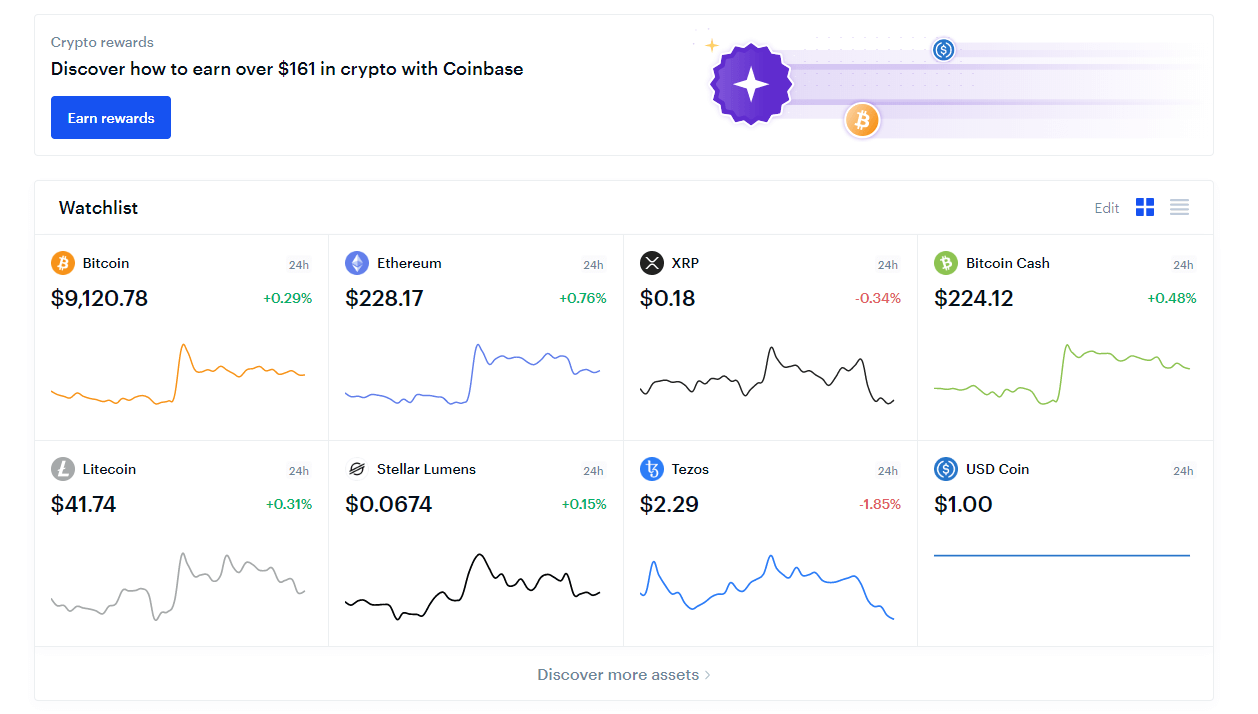The displayed webpage showcases a detailed overview of eight major cryptocurrencies: Bitcoin, Ethereum, XRP, Bitcoin Cash, Litecoin, Stellar Lumens, Tezos, and USD Coin. Each currency is represented with its respective icon against a clean white background. The page features individual graphs illustrating the recent 24-hour activity for each cryptocurrency. Notably, there was a synchronized surge in the value of six cryptocurrencies—Bitcoin, Ethereum, XRP, Bitcoin Cash, Litecoin, and Stellar Lumens—approximately 12 hours prior. Following this sudden spike, the values readjusted and normalized over time. In contrast, Tezos exhibited minimal volatility during this period, and USD Coin maintained a constant value, as it is pegged to the US Dollar.